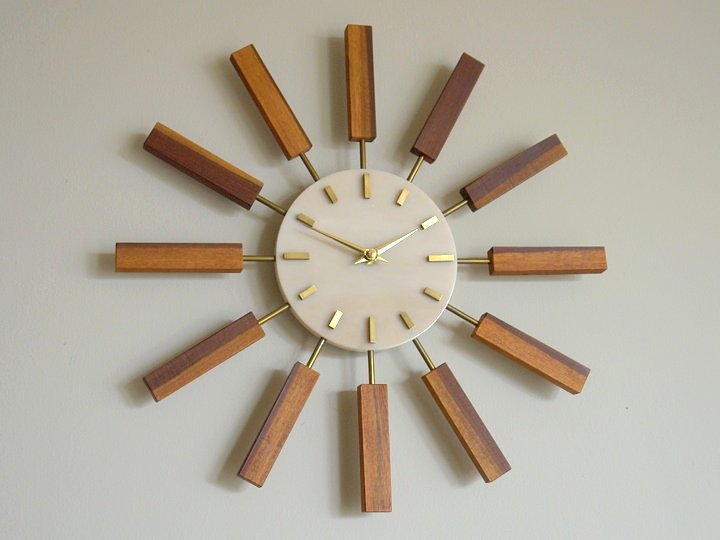The clock is an intriguing and unique design, featuring a central white circle. Unlike traditional clocks, it does not have numbers; instead, the positions for 12, 3, 6, and 9 are marked by gold rectangular blocks. These markers are three-dimensional and slightly larger than the other hour indicators, which share the same design but are shorter and thinner. The clock lacks a second hand, or it might be obscured by the hour hand. Both the hour and minute hands are gold, complementing the aesthetic.

The background of the circular section of the clock has a translucent quality, reminiscent of the material used for Tupperware lids. Extending outward from this central face are gold spokes, each terminating in a rectangular wooden block, effectively marking the hours and adding to the clock's distinctive appearance. Altogether, there are 12 of these extensions, aligning with the hour markers.

This unusual and eye-catching clock is mounted on a beige wall, making it a standout piece in any room.